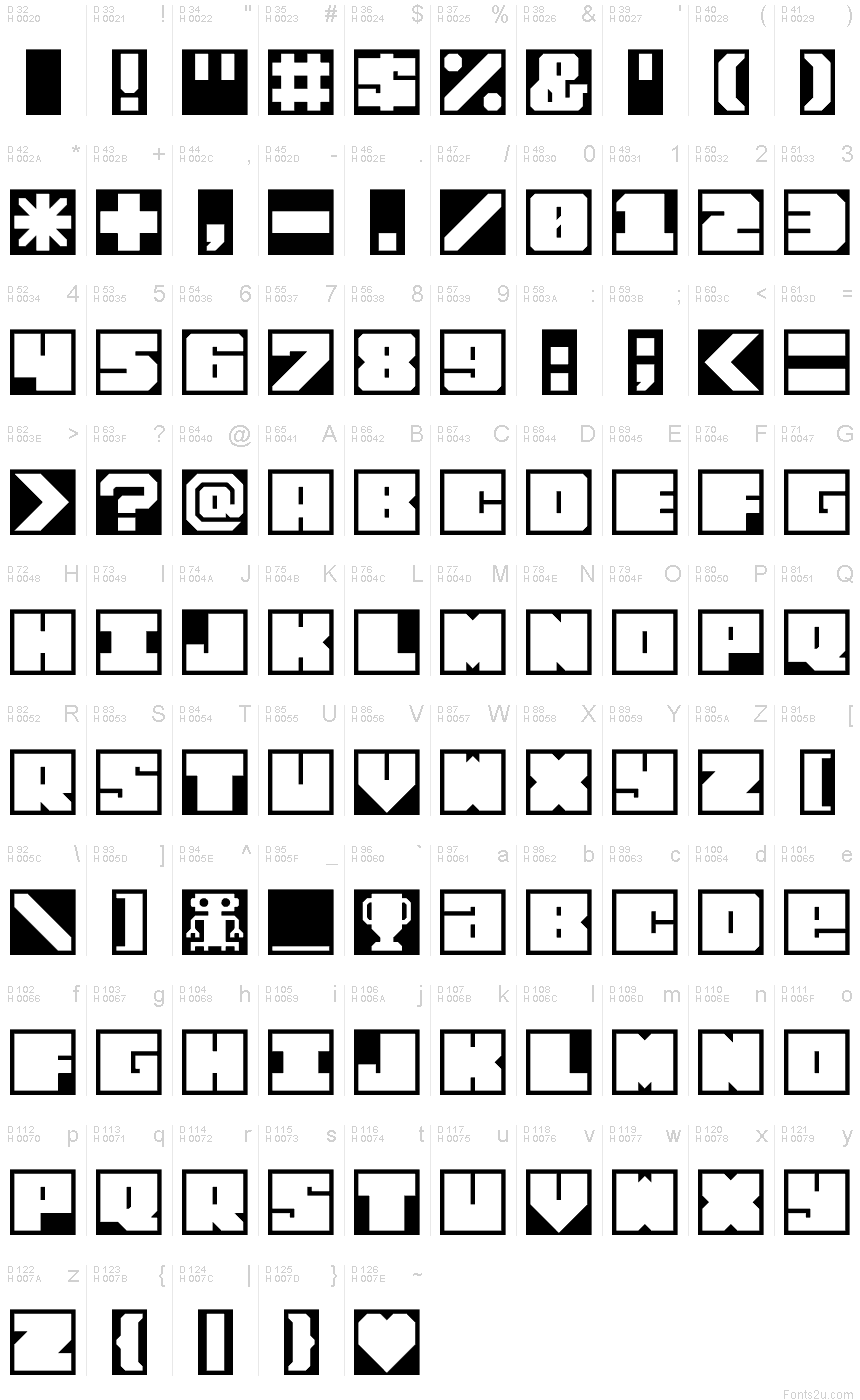This black-and-white image depicts an array of symbols, numbers, and letters organized meticulously into rows, each enclosed within its own distinct box. Above each symbol, number, and letter, there is a header printed in very light gray, detailing specific information such as possible product numbers or ordering codes, though this text is extremely small and largely illegible. A prominent label at the top provides an overarching description of the symbols.

In detail, the array features a diverse collection: recognizable characters like "N," which is explicitly labeled above, suggesting ease of reference or order placement. Among the other symbols, notable ones include a trophy icon, an alien-like figure, and a heart, each distinctly encapsulated in its own box. The background of the image is white, enhancing the contrast between the figures and their outlines.

Symbols, numbers, and letters with a black outline on a white background stand out crisply, while other icons are inversely styled with a white foreground on a black background, ensuring clear visibility. For instance, a number sign (#) and a dollar sign ($) are depicted in white against a black backdrop at the top of the image. This methodical arrangement and contrasting design collectively offer a visually organized and easily navigable display of the various characters.